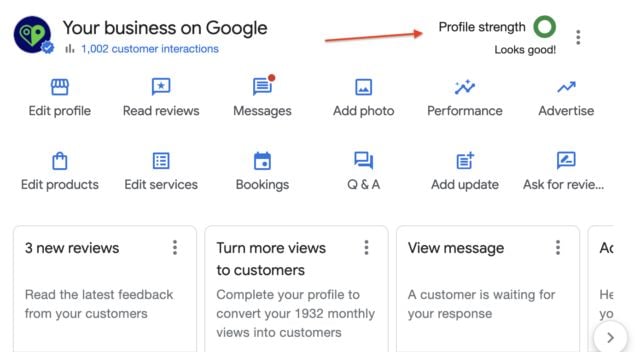In the upper left-hand corner of the image, there is a black text that reads "Your Business on Google." Accompanying this text on the left is a blue circle logo featuring two GPS ping dots, shaped like a heart and angled towards each other. On the upper right-hand side, there's a red arrow pointing at a section labeled "Profile Strength" which is encircled by a green circle with a white center. Beneath this, in smaller font, it reads "Looks Good."

Directly below this section, there are three vertical dots, followed by a series of icons that stretch across the width of the image. Each icon row comprises six icons, making up two complete rows.

Below the icons are three horizontal boxes. The first box indicates "Three New Reviews," the second prompts "Turn More Views to Customers," and the third box reads "View Messages." A horizontal scroll bar is also visible at the bottom of these boxes.